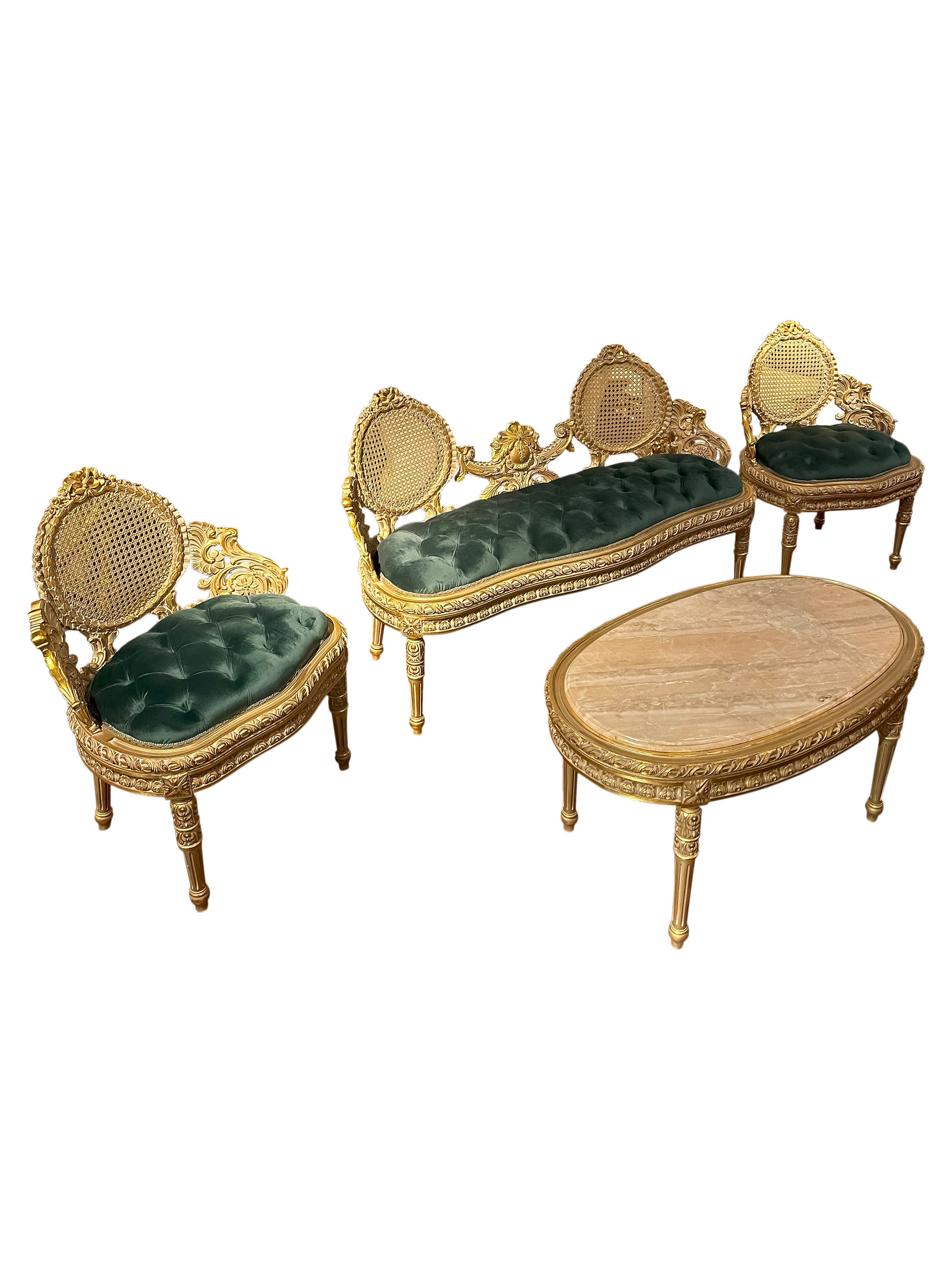The image features a set of ornate, antique-style furniture against a white, minimalist background. The focal points are three single seats and a double settee, all adorned with luxurious green velvet cushion tops, exuding an air of classic elegance. Each piece is lavishly detailed with gold trim, including intricately carved arms and slender legs, enhancing their vintage appeal. The seats display a consistent design theme, characterized by a crisscross pattern in their rounded, gold-framed backs. Complementing the seating arrangement is a low, oval coffee table. The table boasts golden edges and legs, with an opulent tabletop that appears to be light brown or possibly marble, finished to a high gloss. This collection of furniture, with its richly textured fabrics and elaborate gold accents, evokes the grandeur of bygone eras.